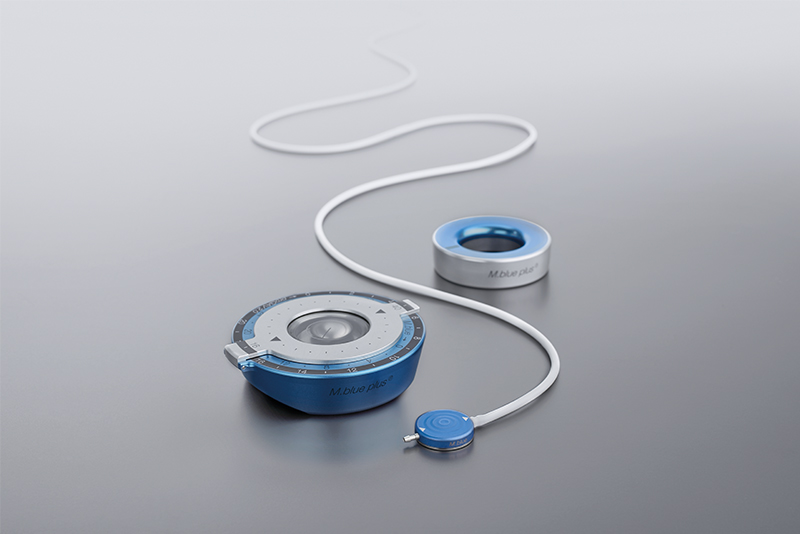This image depicts a detailed, close-up view of a medical device set against a grayish-blue background. The primary subject consists of three distinct components, all made of blue metal and silver-colored materials. One prominent feature is a circular valve with a blue center and a surrounding metal edge, displaying a hole that looks intentionally made. Adjacent to this is a thin white cord running across the image, connected to a small circular blue disc tipped with a metal piece resembling the terminal end of a stethoscope. Another notable element is an item positioned on a blue anodized metal base with a silver top, possibly incorporating a piece of glass in its design, and featuring a series of numbers ranging from 8 to 16 along its edge, indicative of a gauge or dial. The apparatus is identified as a gravitational valve device used for patients with hydrocephalus to manage pressure differentials when changing postures, likely indicating its medical application for addressing posture-related issues in such patients. The side of the image features the text "M Blue Plus," suggesting a model or branding of the medical equipment.